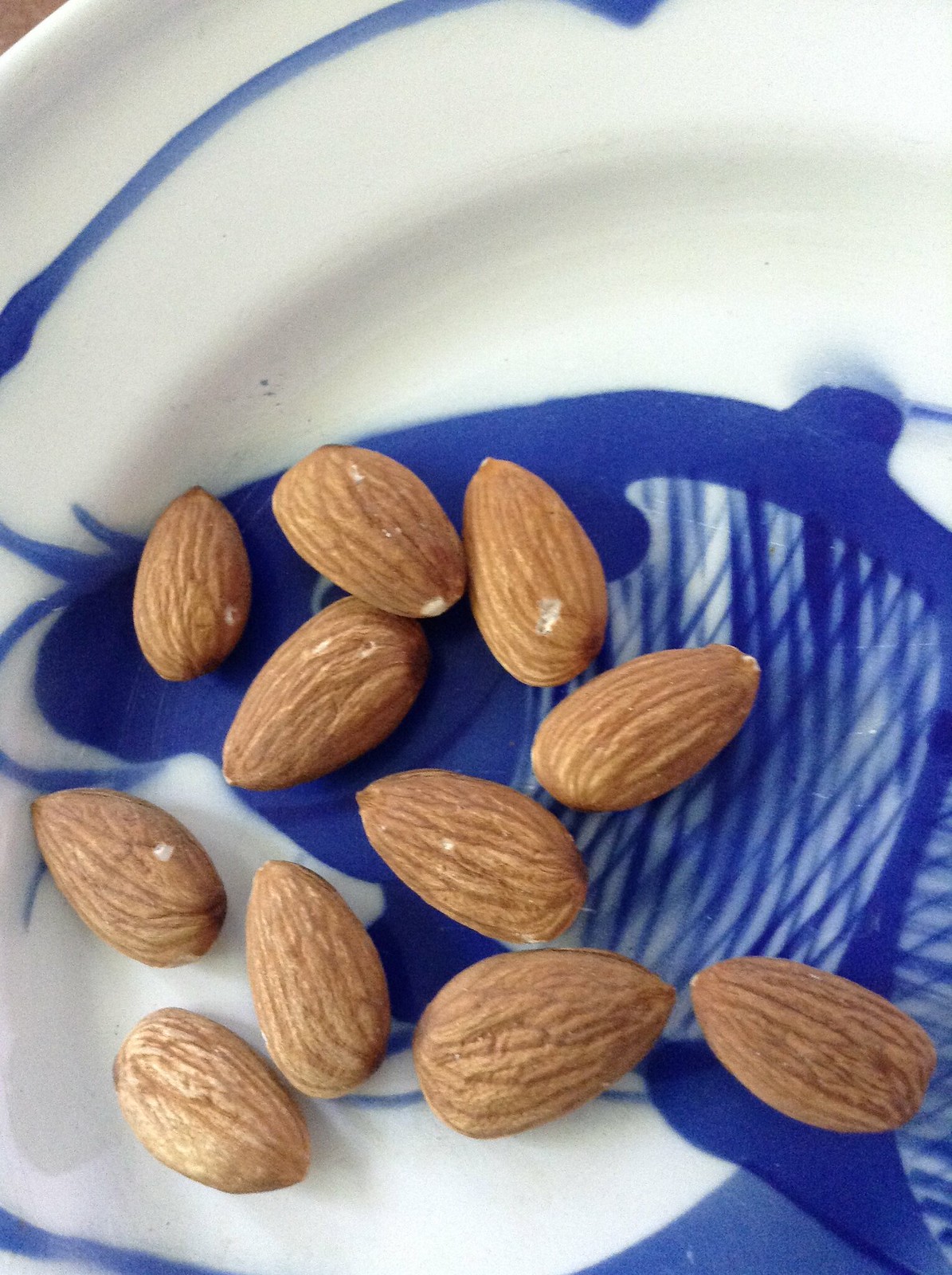The image is a photograph of approximately eleven whole almonds with their skins lying scattered in a dish. The white or cream porcelain dish appears to be hand-painted and features a blue ornamental fish, possibly a koi, with detailed cross-hatching representing its scales. One of the fish's eyes peeks out from between the almonds. The dish is decorated with a blue line around its rim, enhancing its delicate aesthetic. The almonds are unseasoned and randomly oriented, revealing portions of the fish design underneath. There are no utensils or additional items in the image, just the almonds in the artistically designed dish.